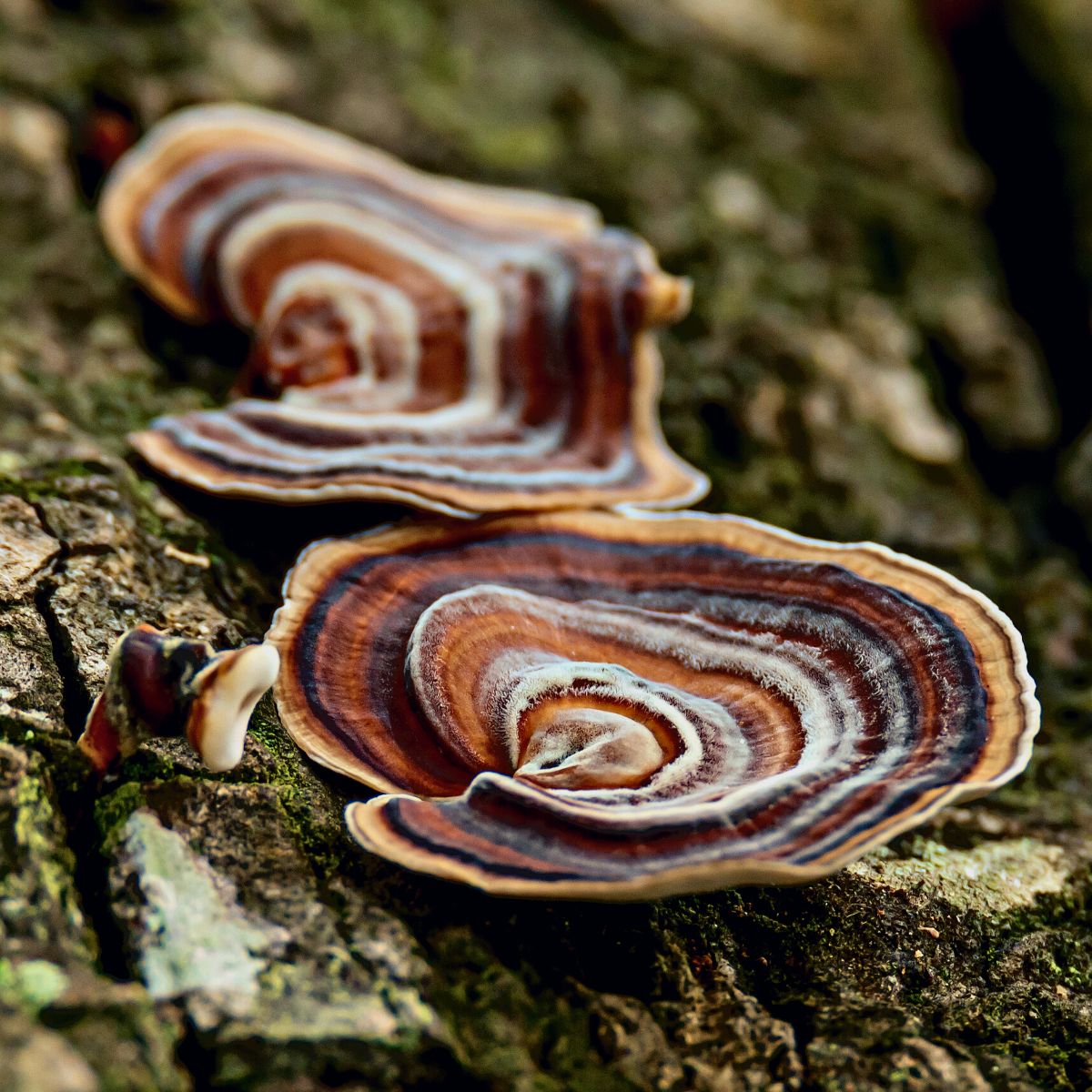In this detailed close-up shot captured outdoors in a forest-like environment, two disc-shaped fungi, vibrant in color, emerge prominently from a wooden surface covered in moss and tree bark. The fungi, situated in the foreground, display concentric rings of orange, white, red, blue, brown, and tan, creating a striking visual against the earthy background. The primary fungus is sharply focused, showcasing its wavy, circular structure, while the secondary fungus in the background appears more distorted and blurred, adding depth to the composition. No animals or people are visible in the image, drawing attention solely to the intricate details of the fungi and the textured bark, both of which occupy the frame's focus. The overall scene conveys a serene, untouched natural setting.